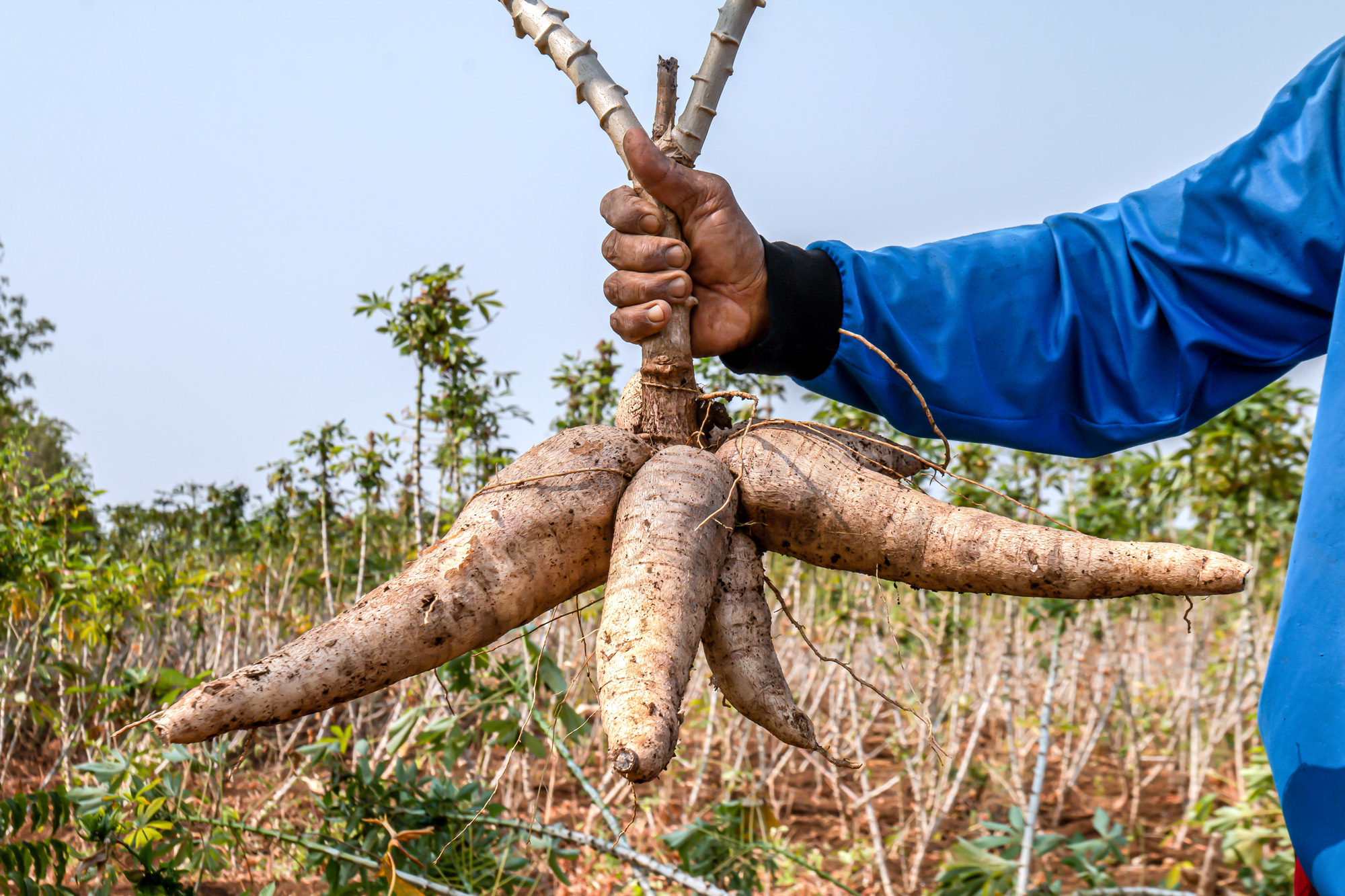The photograph, set in a rural, farm-like environment during daytime, features a man's right arm and hand prominently in the center. The man’s skin is somewhat dark, and his hand appears dirty from working in the field. He is wearing a bright blue, long-sleeved jacket with a dark blue cuff, and the sleeve looks slightly baggy. The hand is grasping a thick, grayish-beige stem, which extends upwards out of the frame and supports a cluster of four root vegetables. These vegetables are elongated, taper at the ends, and are a creamy beige color with small, hairy root structures along their upper edges. They resemble yams or large, light-brown potatoes. Behind the man, the background reveals a field filled with various plants and long growth, interspersed with brown grass, contributing to the rustic and agricultural atmosphere of the scene.